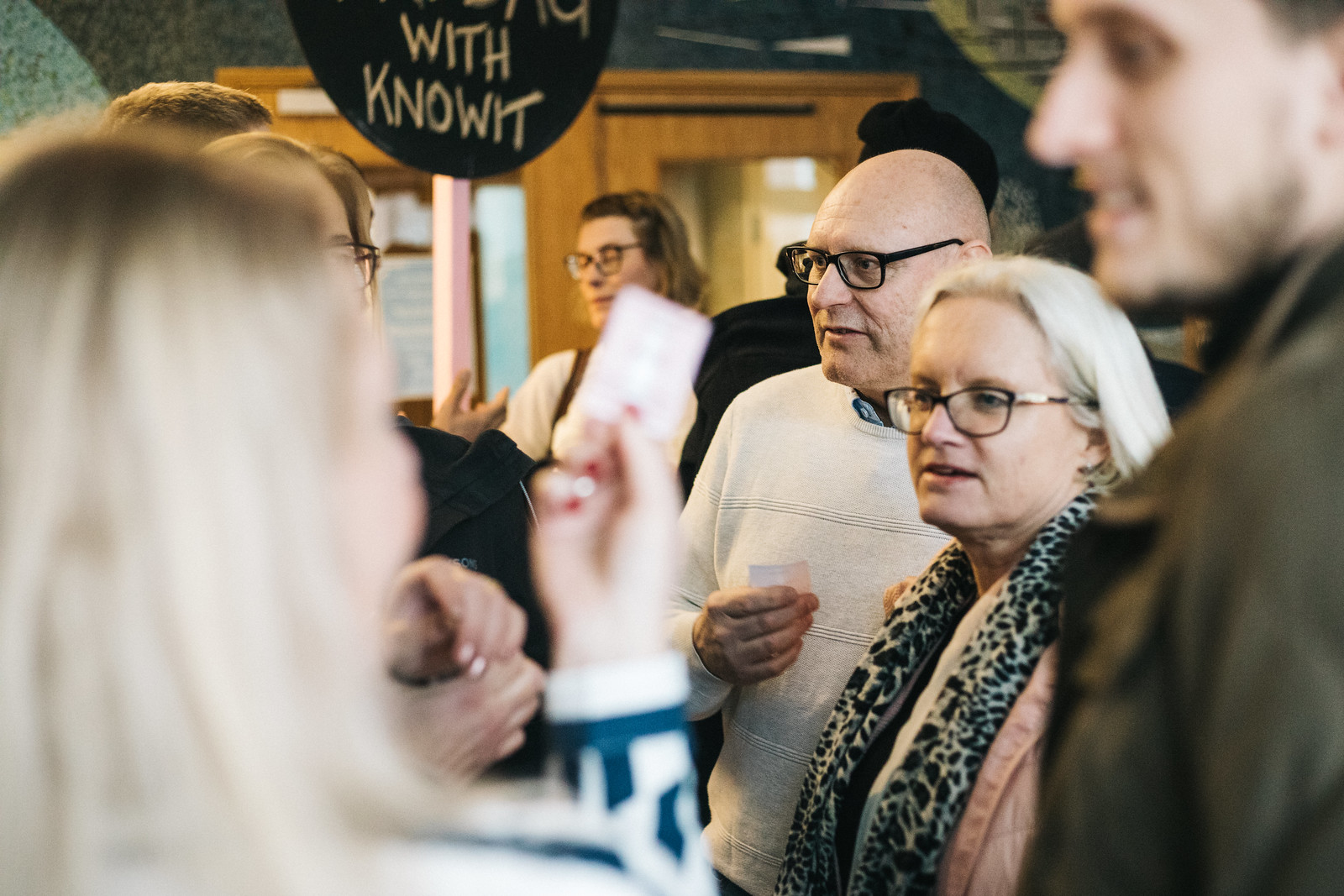The photograph features a group of middle-aged to older individuals gathered in a room, engaging in conversation and mingling. In the foreground, the main focus is on a bald man and a woman, both wearing glasses. The man, clad in a whiteish-tan knit sweater with lines, holds a white piece of paper in his right hand. Next to him, the woman sports a pinkish coat and a black-and-white leopard print scarf, also donning black eyeglasses. She appears to be conversing with others around her. Among the crowd, there are additional individuals visible, some holding papers, and another woman on the left who is also holding up a piece of paper, though it is blurry. In the background, a noticeable black circular sign with white and yellow writing at the bottom reads, "With Knoweth." This sign seems to be part of the event, although the exact context or purpose of the gathering is unclear.